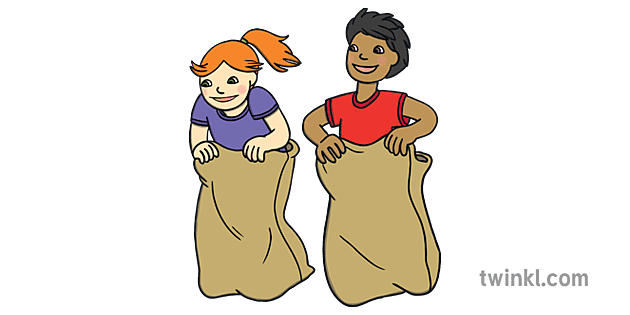This animated, computer-generated image depicts two children in the middle of a potato sack race set against a plain white background. The girl on the left, distinguished by her fair skin, light red or orange hair tied in a ponytail with bangs, and sporting a cheerful expression with light pink cheeks, is wearing a short-sleeved blue (or possibly purple) shirt and clutching her burlap sack with both hands in front of her. To her right is a tan-skinned child, with short black hair and brown eyes, dressed in a red shirt. This child is also smiling and holding their potato sack similarly with both hands. Both figures exhibit simplified, cartoonish facial features, characteristic of children's book or TV show illustrations. The playful scene is accompanied by the text "twinkl.com" in gray font, located at the bottom right corner of the image. The overall atmosphere suggests a fun and lighthearted event between the two participants.